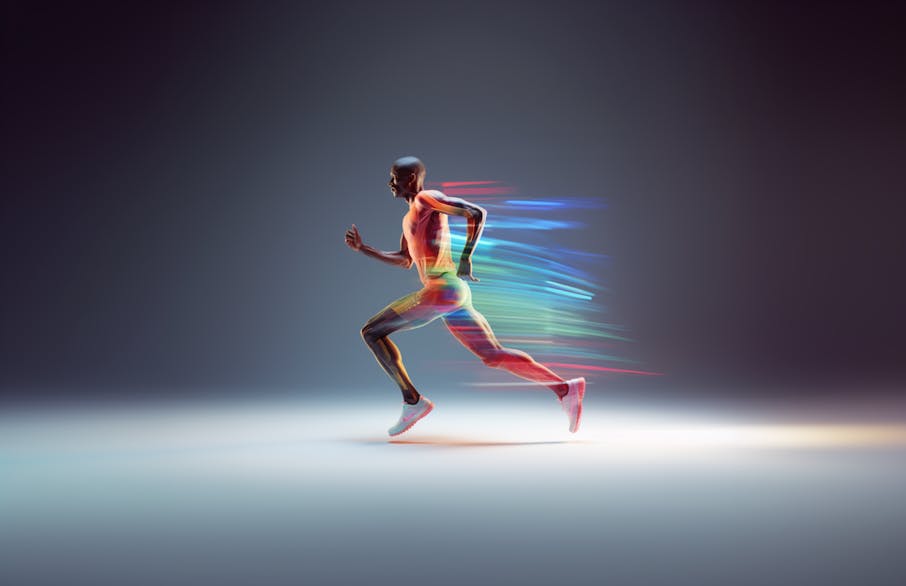In this stylized image, an African-American man with a closely shaved head is depicted in dynamic motion, running towards the left side of the frame. The background features a dark gray hue that gradually fades to white near the bottom, giving the impression of a staged set rather than an outdoor scene. The runner's attire is a vibrant, rainbow-colored unitard that appears superimposed with strikingly vivid blues, purples, and oranges, accentuating his movement and speed. His right arm is extended forward while his left arm is bent back, and his left leg is thrust ahead with his right leg trailing behind, toes just off the ground. Special effects, including lines, waves, and blurs of light, emanate from behind him, emphasizing his rapid pace as if he were creating wind. The lighting suggests an indoor studio environment, highlighting the runner's form and the kinetic energy around him. His white sneakers feature distinctive pink accents on the bottoms and a unique design on the side, enhancing the overall impression of swift, powerful motion.